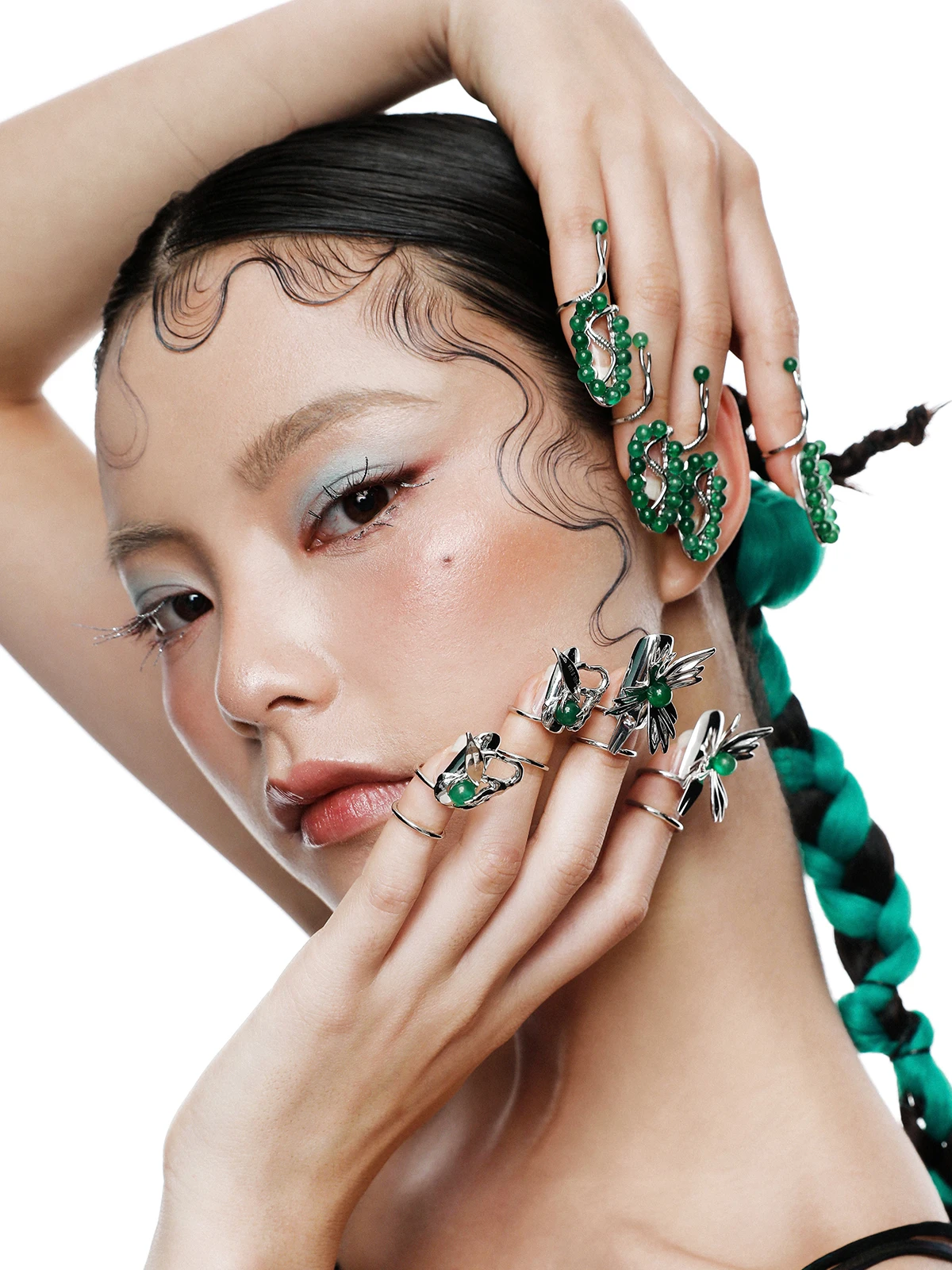The image features an Asian woman standing against a white background with possibly photoshopped elements. She has her black hair pulled back tightly into a low ponytail, interwoven with a green ribbon. Thin strands of hair rest along the sides of her face, styled to create a ruffled effect. Her facial features include thin eyebrows, long eyelashes, and blue eyeshadow. She poses with one hand over her head and the other resting on her cheek, displaying a range of unique silver rings on every finger. The rings on one hand are thin wire designs with small green beads forming a circular pattern, while the rings on the other hand resemble small butterflies with a single green bead in each. She wears a black dress, just visible at the shoulder, and looks directly into the camera.